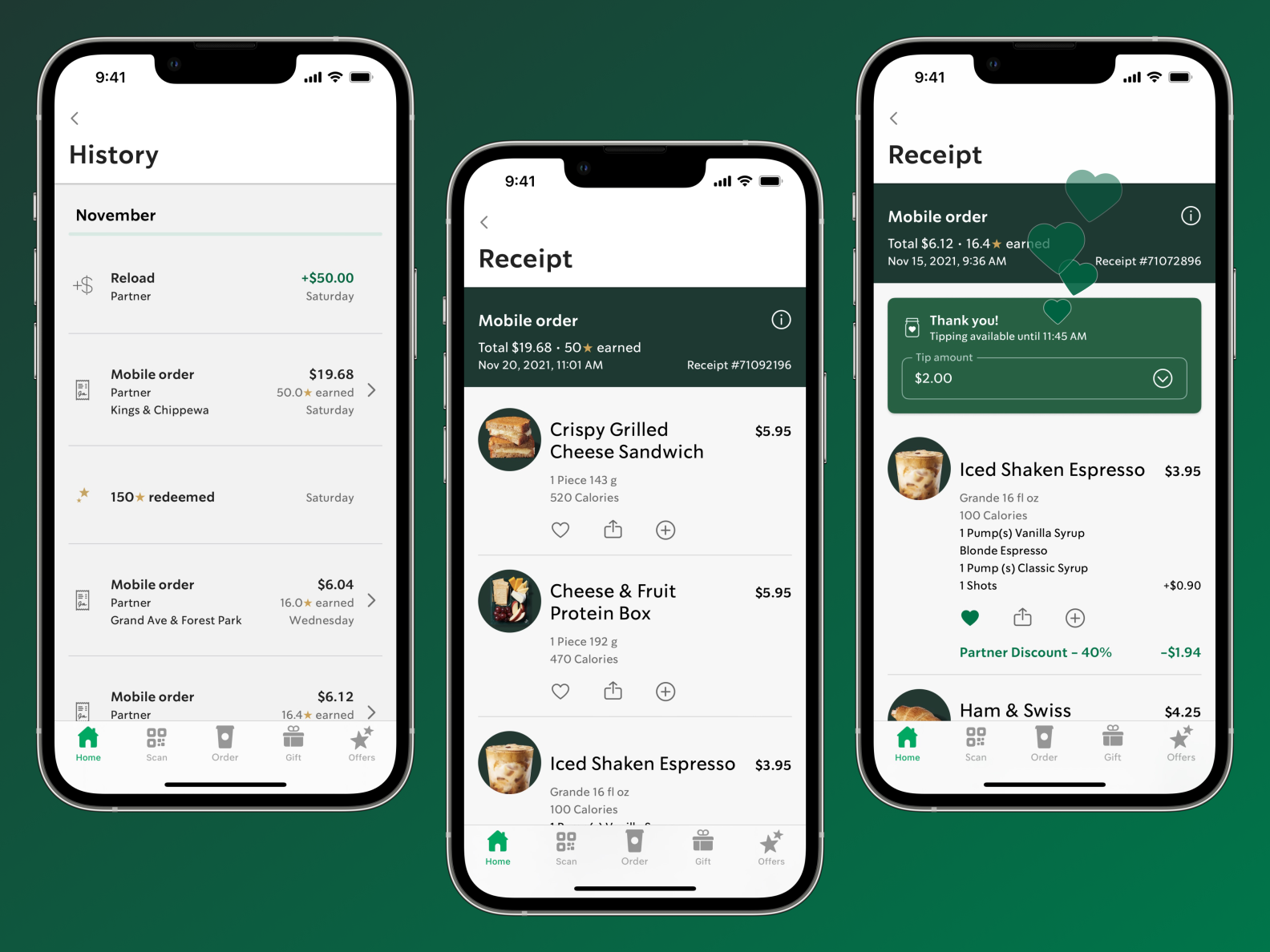**Concept Design for Mobile Ordering App**

The image showcases a conceptual design for a mobile ordering app, beautifully presented against a gradient green background that transitions from a light shade at the bottom to a darker hue at the top. The layout consists of three mobile phone screens, with the first and last phone positioned higher, and the middle phone slightly lower, creating an approximate 80% overlap among them for a dynamic, staggered effect.

The first phone screen displays a "History" page detailing a user's past orders and actions, organized into six distinct rows with a gray background and horizontal dividing lines. The history pertains to November and includes:

1. **Reload Partner** - An action of adding $50 on Saturday.
2. **Mobile Order at Partner Kings and Chippewa** - An order costing $19.68, earning 50 stars on Saturday.
3. **150 Stars Redeemed** - Gold five-point star, happening on Saturday.
4. **Mobile Order at Partner Grand Ave and Forest Park** - An order costing $6.04, earning 16 stars on Wednesday.
5. **Mobile Order** (partially cut off) - Costing $6.12 with 14.6 stars earned.

At the bottom of each phone screen are five icons: Home (highlighted in blue), Scan, Order, Gift, and Offers. Each icon has a distinct symbol above it: 

- Scan features a 2x2 grid with the fourth box containing another grid.
- Order presents a white circle in the center.
- Gift displays a present.
- Offers shows two stars, with the second star being smaller and positioned to the upper right.

The middle phone screen shows a detailed "Receipts" page for a specific mobile order:

- A green bar at the top displays the total amount ($19.68), stars earned (50), date (Nov 20, 2021), time (11:01 AM), and receipt number in white text. 
- Beneath the total, there's a summary of ordered items, each illustrated with pictures inside green circles: a crispy grilled cheese sandwich, a cheese and fruit protein box, and an iced shaken espresso.

The final phone screen also displays a "Receipts" page similar to the middle one but includes additional details:

- A forest green box at the bottom features a “Thank You” message, with a tip amount of $2 and hearts emanating vertically like smoke.
- The specific items listed include an iced shaken espresso and, partially visible, a ham and Swiss sandwich.

This conceptual design effectively showcases the app's user interface and functionality, emphasizing ease of navigation and detailed transaction history.